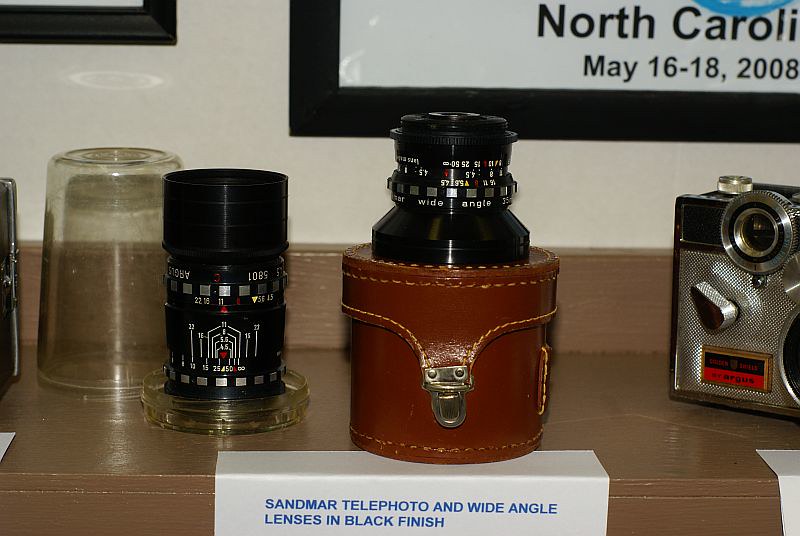In this indoor, full-color photograph, a wooden shelf is neatly organized with various vintage camera equipment against an off-white wall. The primary focus is a collection of old camera parts. Dominating the scene, centered on the shelf, is a white piece of paper that prominently displays the text "Sanmar, Telephoto, and Wide Angle Lenses in Black Finish." This paper is partially held down by a brown leather cylindrical case on its right, which is designed to store camera lenses. Beneath this case hangs a small plaque bearing the same text as on the paper.

To the right of the leather case, there is a partially visible vintage Argus camera. This camera is characterized by a silver, textured body, featuring a distinctive black and red square logo with a small shield that reads "Golden Shield." The camera includes a triangular silver handle and a half-visible silver knob. Part of the lens and the photo-taking button are also visible.

On the left side of the leather case, there's a smaller camera lens with visible markings, likely for lens adjustments. Further to the left, there's a glass cup turned upside down, and next to it, another tall camera lens—with its lens cap placed underneath it, likely because the original cap was lost. 

Above the shelf, a black-framed photograph hangs on the wall, with the text "North Carolina, May 16th through the 18th, 2008" clearly inscribed. There's also the edge of another photo frame peeking in from the top left corner of the image. The black frame and the off-white wall provide a contrasting background to the vintage items displayed on the wooden shelf.